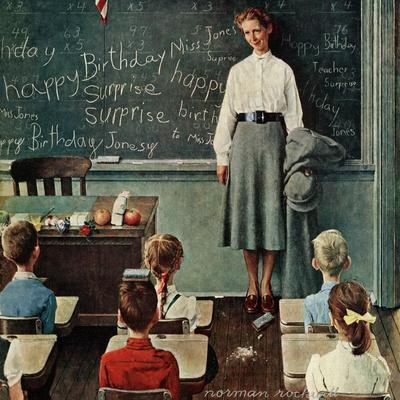The image depicts a classic 1950s-style classroom, characteristic of a Norman Rockwell painting. It features a teacher, Miss Jones, standing in front of six desks occupied by a diverse group of boys and girls. The two desks on the far left are partially visible with students seated behind them. The teacher, dressed in a white, long-sleeved blouse cinched with a broad black belt and a gray skirt that extends below her knees, stands at the front of the room. She holds a jacket and a white hat in her left hand and directs a jubilant smile towards a student sitting in the middle, who playfully balances books on his head. The chalkboard behind her is adorned with affectionate messages like "Happy Birthday Miss Jones" and "Surprise, surprise," revealing that the scene captures the moment Miss Jones is greeted with a birthday surprise from her students. On the floor before her, a piece of chalk and an eraser lie amid a small cloud of chalk dust, adding a casual touch to the setting. A robust wooden desk to her left is laden with two apples and what appears to be a box containing a gift, completing this heartwarming and nostalgic portrayal of a mid-20th century American classroom.